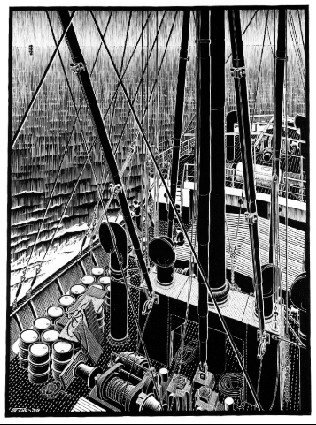This black-and-white illustration, titled "Freighter" by M.C. Escher, created in 1936, is a highly detailed line art sketch of a large sailing vessel. The ship, positioned centrally and dominating the portrait-oriented image, showcases a myriad of intricate elements. A prominent mast stands towards the right third of the composition, anchored into a horizontal deck structure and surrounded by numerous stacked barrels. The deck is interwoven with ropes and cables stretching in various directions, indicating a complex rigging system likely related to sails or an anvil-crank mechanism. The vessel's railing is visible along the sides and near the front, although the precise contents at the bow are indistinct. Below the ship, intense rippling waters suggest a torrential downpour, with rain depicted as straight, forceful lines adding to the dramatic atmosphere. The scene, framed by a black border, is set outdoors on an ocean, with a lighter horizon line glimpsed at the image's top. The entire composition, rendered solely in shades of black, white, and gray, exemplifies modern art illustration techniques.